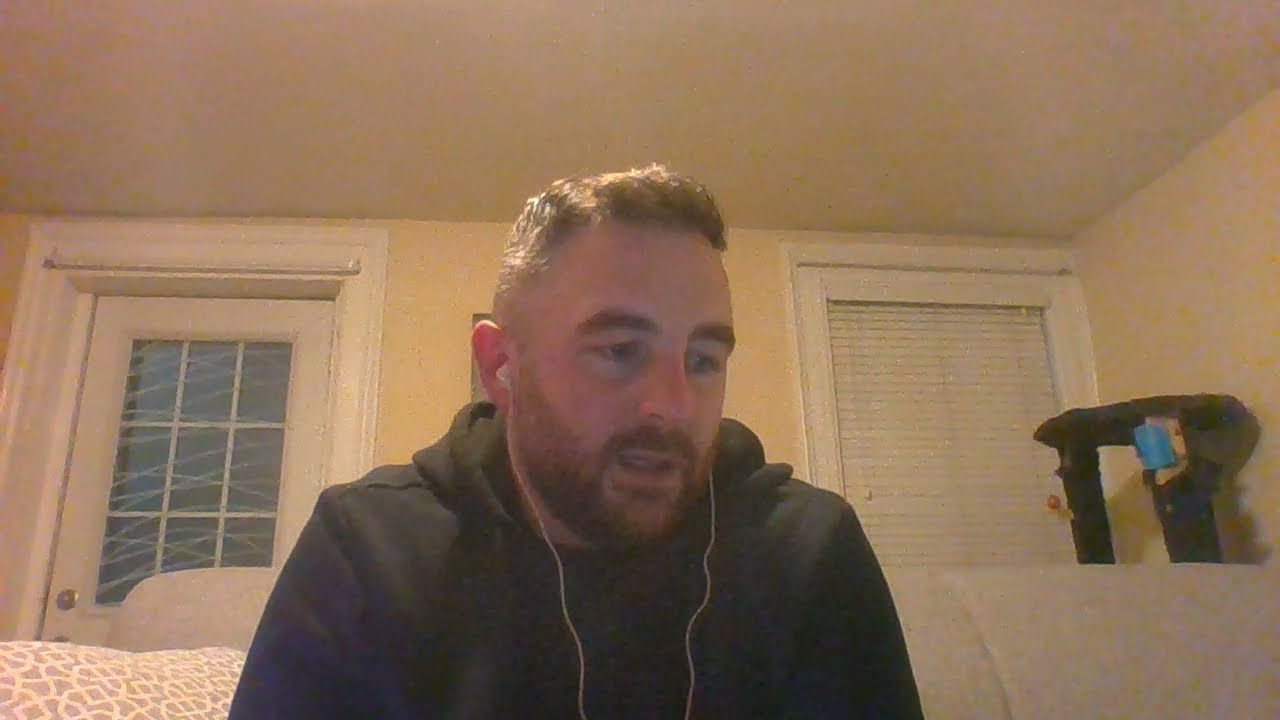The photograph captures a middle-aged white man seated on a white or cream-colored couch in an indoor setting. He is wearing a black or dark gray hooded sweatshirt and white earbuds with wires. The man has light brown, short hair, particularly trimmed on the lower sides, bushy eyebrows, and a full, trimmed beard and mustache. His gaze is directed downward. Behind him, the wall is a light yellow color with white-trimmed fixtures, featuring a door on the left and a window on the right. There is also an indistinct object with bars or a plastic structure to the right behind the couch. The camera angle is positioned at the man's chest level, slightly angled upwards towards his face, framing the indoor setting and emphasizing the couch.